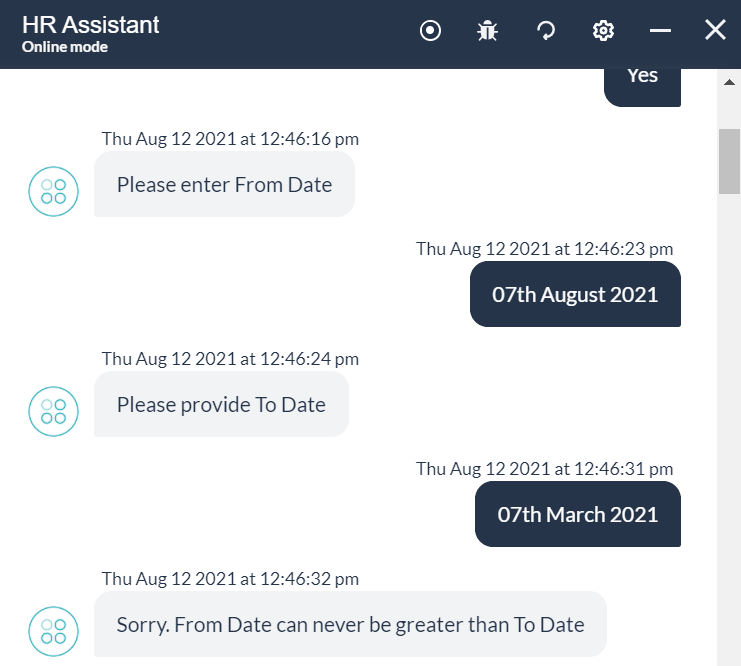The image depicts a user interface of an AI chat assistant found on a webpage. At the top of the chat window, there's a navy blue bar with "HR ASSISTANT" written in white, indicating the functionality of the chatbot. Below this, in smaller text, it reads "Online Mode," illustrating the bot’s availability status.

To the right side of this navy blue bar, there are several symbols: a circle with a solid white dot in the center, followed by a small bug icon, an arrow forming a half-circle, a settings gear icon, a dash line, and an "X" for closing the chat. These icons likely represent various functionalities like notifications, bug reporting, refresh, settings, minimize, and close, respectively.

The chat interface itself has a dark blue background for the user's messages and a dark gray background for the chatbot's responses. In the conversation shown, the user’s first message simply states "Yes." The chatbot, identified by a symbol of four small circles arranged into a square, prompts the user to "Please enter date." The user then inputs "07 August 2021." The bot replies asking for the "to date," to which the user responds with "07 March 2021." The bot then issues an error message stating, "Sorry, from date can never be greater than to date."

The layout and symbology of the interface are clean and indicative of standard design practices for interactive AI chat assistants.